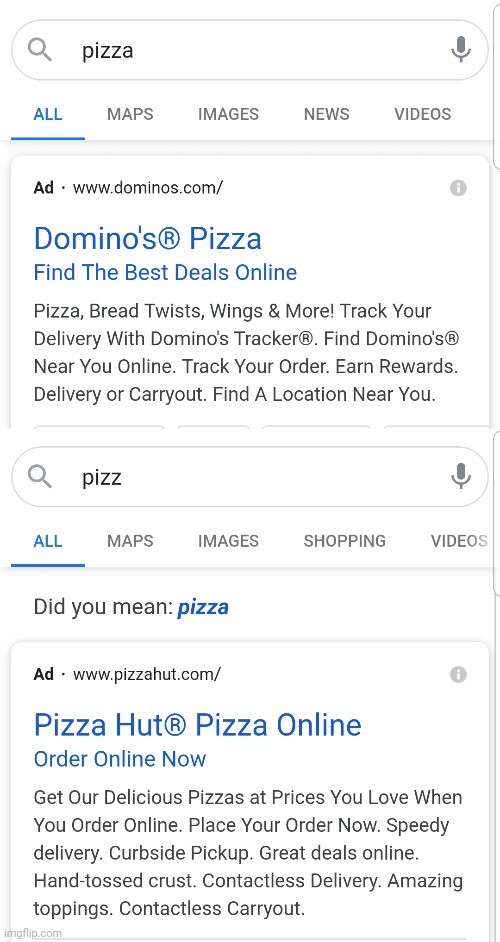Title: Detailed Screenshot Analysis of Pizza Search Results

Caption: The screenshot captures a web search focused on pizza. At the top, the browser's navigation bar displays tabs for 'All,' 'Maps,' 'Images,' and 'News.' The first search result is an advertisement for Domino's Pizza, prominently featuring a clickable blue link reading "Domino's Pizza." The ad highlights various offerings such as pizzas, bread twists, wings, and more, and mentions the ability to track your delivery.

Directly below, another search bar shows the partially typed term "P-I-Z-Z" with autocomplete suggestions. Right underneath the search bar, a prompt asks, “Did you mean pizza?” The search tabs available in this section include 'All,' 'Maps,' 'Images,' 'Shopping,' and an icon for voice search.

Following this, another advertisement appears for Pizza Hut, promoting online ordering. It emphasizes delicious pizzas at favorable prices, speedy delivery, curbside pickup, and exclusive online deals.

The image source is identified as imageflip.com. The structure of the screenshot repeats with another search result for Domino's Pizza, including similar elements such as the search bar, suggestion prompt, and the navigation tabs. The recurring ads and search elements emphasize pizza-related promotions and deals from Domino's Pizza and Pizza Hut.